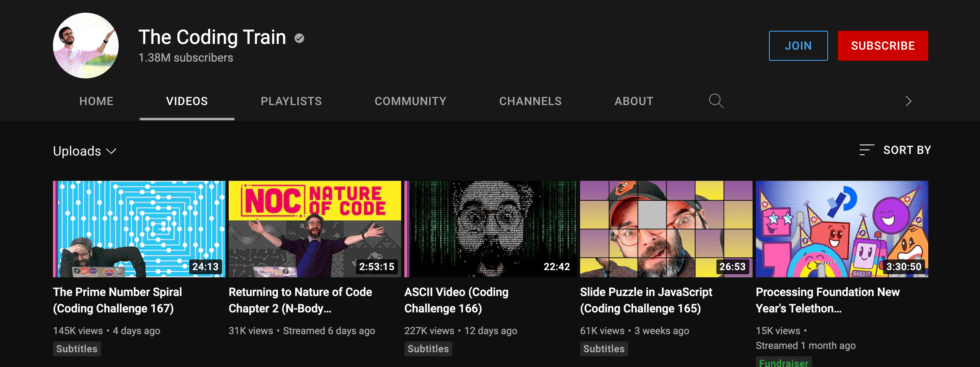The image shows a YouTube page named "Decoding Train," which is a verified channel with 1.38 million subscribers. The page is set against a black background. The upper left corner features the channel's name and a profile icon depicting a person in a pink t-shirt raising their right hand. On the top right of the page are two buttons: a red "Subscribe" button and a blue "Join" button beside it.

Below the channel name, there are several tabs: Home, Videos, Playlists, Community, Channels, About, and a Search icon. The "Videos" tab is currently highlighted in white, while the other tabs are shown in grey. Underneath the "Videos" tab, there is an "Upload" drop-down menu. 

The video section displays five videos:
1. "The Prime Number Spiral Coding Challenge 167" with 145k views, uploaded four days ago. This video includes subtitles.
2. "Returning to Nature of Code - Chapter 2" with 31k views, streamed six days ago. 
3. "ASCII Video Coding Challenge 166" with 227,000 views, uploaded 12 days ago. This video also includes subtitles.
4. "Slide Puzzle in JavaScript - Coding Challenge 165" with 61k views, uploaded three weeks ago. This video includes subtitles as well.
5. "Processing Foundation New Year's Telethon," which has 15k views and was streamed one month ago. This video is marked as a fundraiser, indicated in grey text.